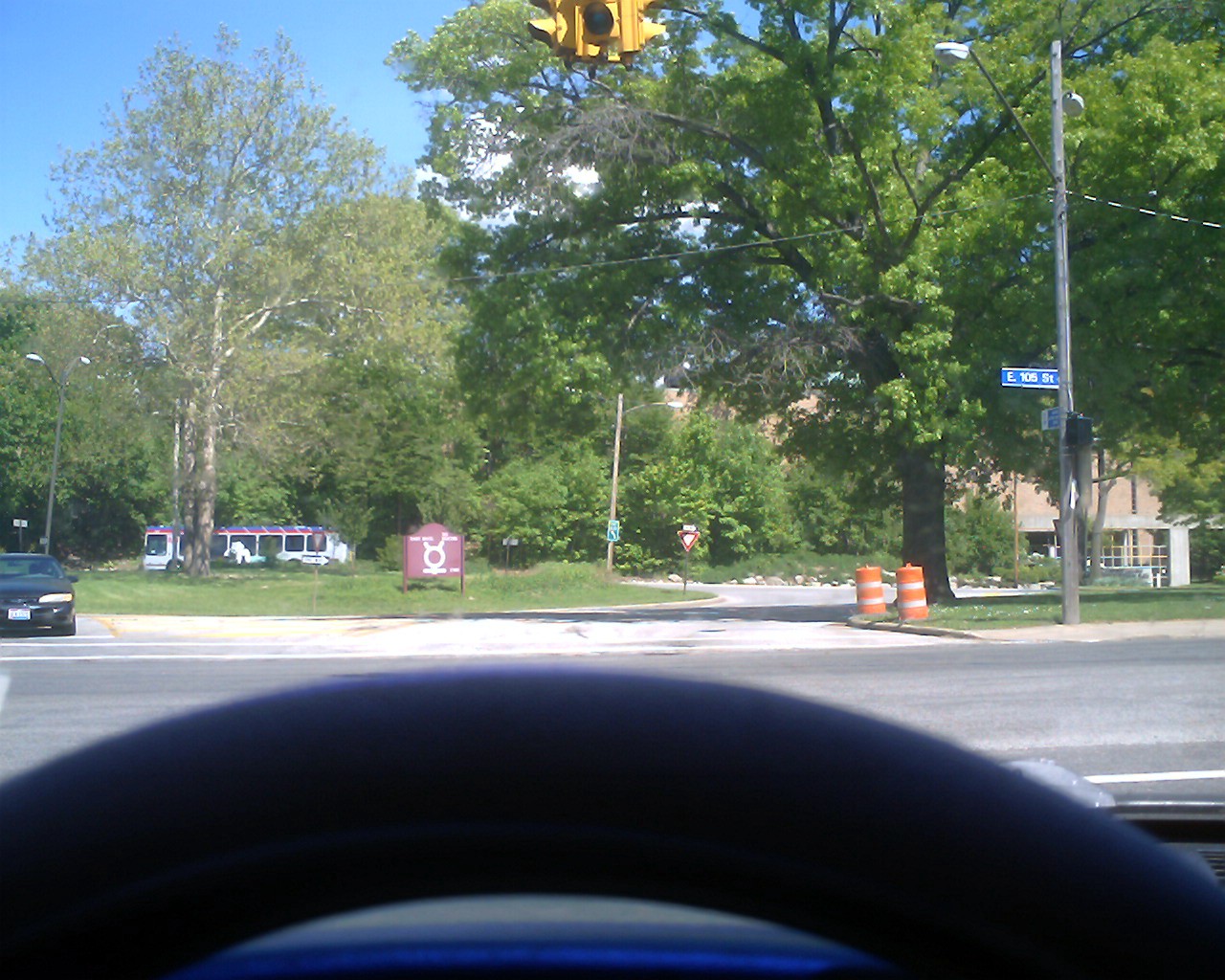The image depicts a detailed view through a car's windscreen, capturing the top edge of a black steering wheel and a dashboard tinged with a hint of blue from an illuminated LED panel or ambient light. Beyond the windowpane, a parallel road is visible, featuring another car stationed on the opposite side, likely poised to turn at the junction. On the right stands a telegraph pole adorned with a small blue sign and overhead lights, contributing to the street's illumination. Central to the scene, yellow traffic lights are oriented west, east, and south, directing traffic from multiple angles. The backdrop reveals numerous trays and a few buildings, adding depth and context to the urban surroundings.